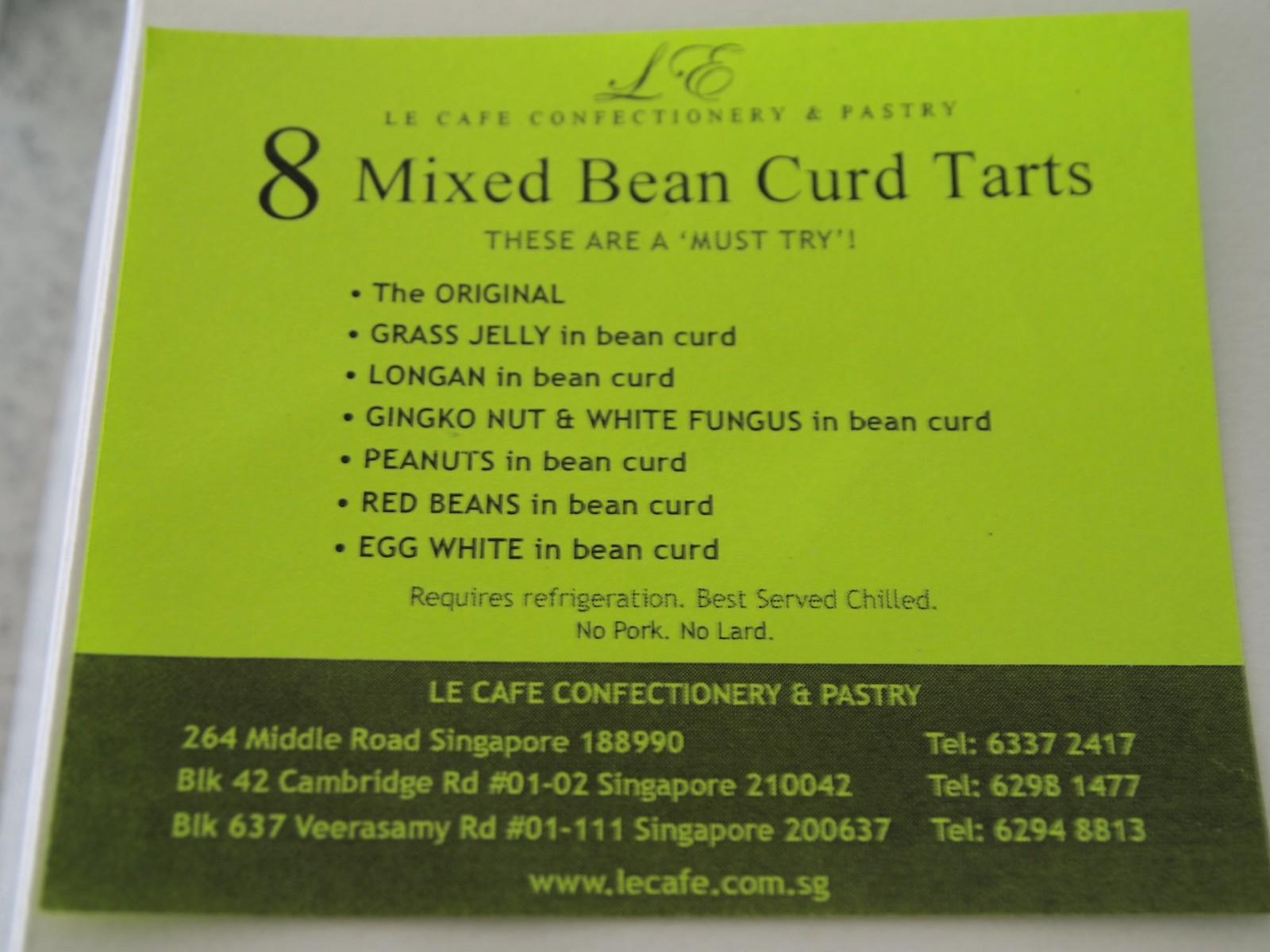The image is of a vibrant neon green card from Le Café Confectionary and Pastry, promoting their Eight Mixed Bean Curd Tarts. The top two-thirds of the card, in neon green, features the café's logo in cursive with the letters "L" and "E" prominently displayed. Directly below, in black text, is the name "Le Café Confectionary and Pastry." Large text highlights the offering: "Eight Mixed Bean Curd Tarts," followed by a smaller, all-caps note that reads "These Are A Must Try." The card lists the different flavors of tarts in a bulleted format: the original, grass jelly and bean curd, longan and bean curd, ginkgo nut and white fungus and bean curd, peanuts and bean curd, red beans and bean curd, and egg white and bean curd. Additional small text at the bottom of the neon green area states, "Requires Refrigeration, Best Served Chilled, No Pork, No Lard." The bottom third of the card features a black banner with neon green text, repeating "Le Café Confectionary and Pastry" along with three addresses and phone numbers: 264 Middle Road, Singapore, 188990 (6337-2417), BLK 42 Cambridge Road, 01-02 Singapore, 210042 (6298-1477), and BLK 637 Virasami Road, 01-111 Singapore, 200637 (6294-8813). The café's website, www.lecafé.com.sg, is listed at the very bottom.